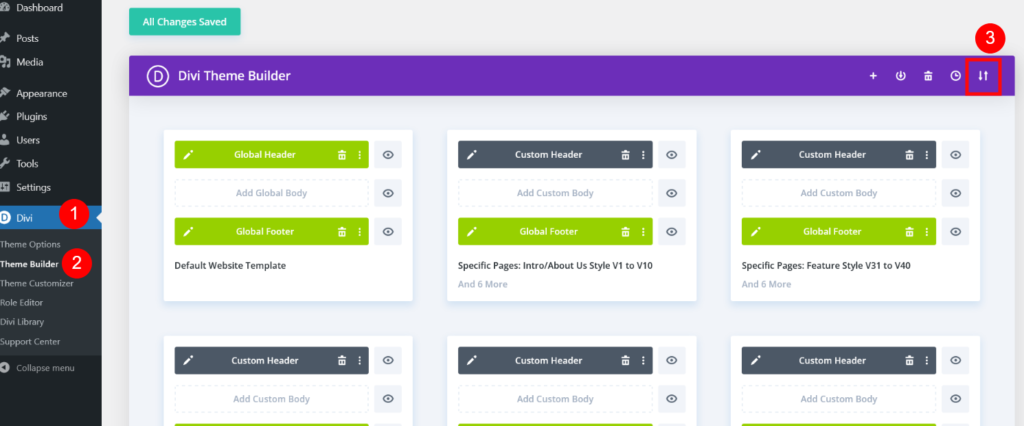The screenshot displays a comprehensive view of a WordPress management interface, highlighting various elements essential for website design and customization using the Divi Theme Builder. 

On the left side of the screen, the sidebar lists the main navigation options: Dashboard, Posts, Media, Appearance, Plugins, Users, Tools, Settings, among other features. 

To the right, the main section showcases the actual website preview. At the top, there is an aqua green notification bar that reads "All Changes Saved." Beneath it lies a purple banner labeled "Divi Theme Builder" accompanied by various options on the right side, including toggles to enable or disable settings. Additionally, there is a circle icon divided into an up and down area, featuring the number three and a logo, whose precise function is unclear.

Below this, the interface is segmented into three rectangular sections. The first section is labeled "Global" and includes options such as "Global Header," "Add Global Body," and "Global Footer". Each of these elements allows for site-wide adjustments and customizations.

The middle section covers the "Default Website Template," offering spaces for "Custom Header," "Custom Body," and "Custom Footer," permitting distinct designs for different areas of the website. It also mentions various specific pages like "Intro," "About," and "Style," and provides an option to add six more customized pages.

The third section, on the right, also provides options for settings related to the "Custom Header." This entire layout facilitates the detailed customization of various aspects of the website, enabling users to configure headers, footers, and body content according to their preference.